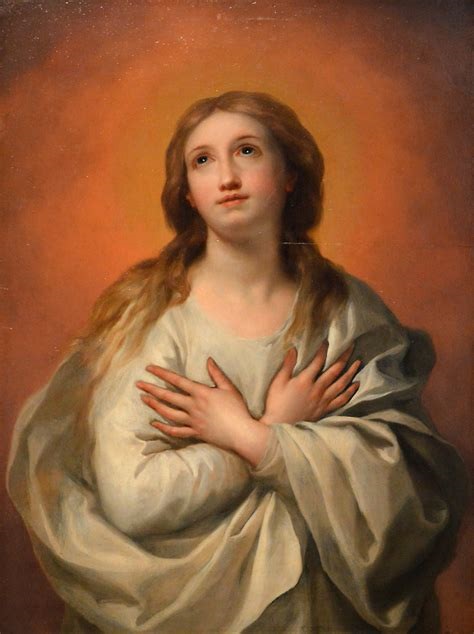The image depicts a beautifully painted portrait of a woman with a pensive expression, as if she is in prayer or deep contemplation. The background is a mix of brownish-orange hues, with darker shades toward the corners, giving the effect of an aura or glow behind her. She has long wavy brown hair that falls to her shoulders and striking blue eyes that gaze upward toward the top of the image. Her cheeks have a peachy color that adds a touch of warmth to her face. The woman is adorned in a white shirt that features a brown collar, and she wears a very long scarf or robe over it. Her hands are crossed over her chest, emphasizing her serene and introspective demeanor.